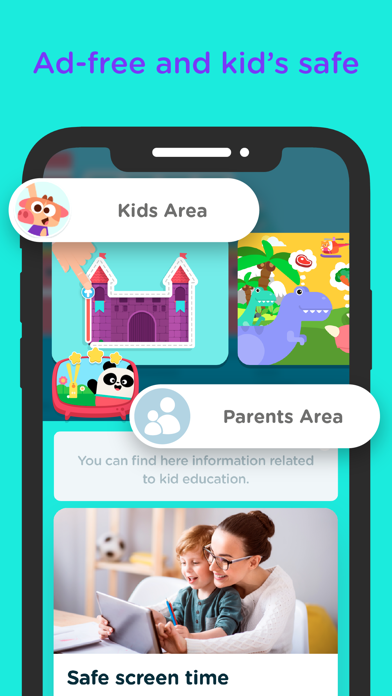The image is a promotional screenshot for a new app. At the top, in a vibrant violet-blue font, it boasts the features "Ad-free" and "Kids-safe." Below this, there is a simple line drawing of a smartphone. Prominently displayed on the phone is a 3D-like button labeled "Kids Area," accompanied by a whimsical cartoon giraffe character. Another tab labeled "Parents Area" is situated below, indicating that users can find information related to child education here. The screenshot includes a preview of an article within the app, featuring a woman holding a child around the ages of 5 or 6, both focused on a tablet. At the bottom of this section, the article title "Save Screen Time" is displayed in bold black text.